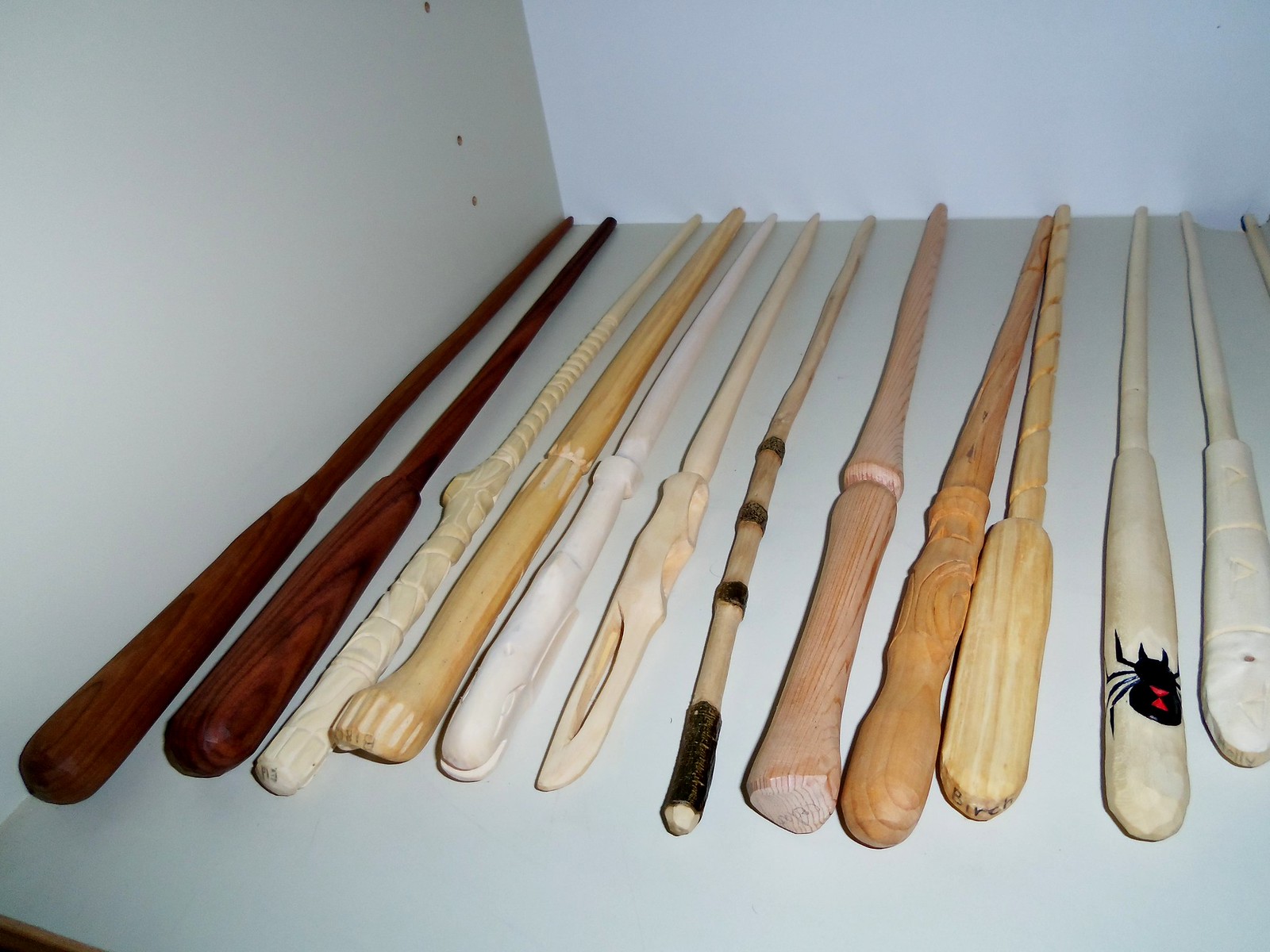The image showcases an assortment of intricately crafted wooden wands laid out on a white surface, likely encased within a white box or shelf, as evidenced by the visible side and back walls. The wands vary widely in color, texture, and design, presenting a rich visual tapestry. Starting from the left, there are two dark wood wands, followed by one of lighter wood. Next to these is a medium-toned wand, succeeded by a very white wand, and then a lighter wood piece. One of the wands has strings artistically wrapped around its handle. Among these is also a wand with a black handle, contributing to the assortment's visual diversity. Notably, the collection includes a wand with a knife-like handle, adding to the variety in thickness and style. Each wand carries unique carvings and details, from carved white staffs to light wood wands with intricate patterns. Additionally, there is a driftwood-like staff with a slight bend and dark markings at the bottom. One particularly thicker wand features a carving in its middle, while another white wand displays a distinctive black spider or black widow symbol, enriching the ensemble’s character.